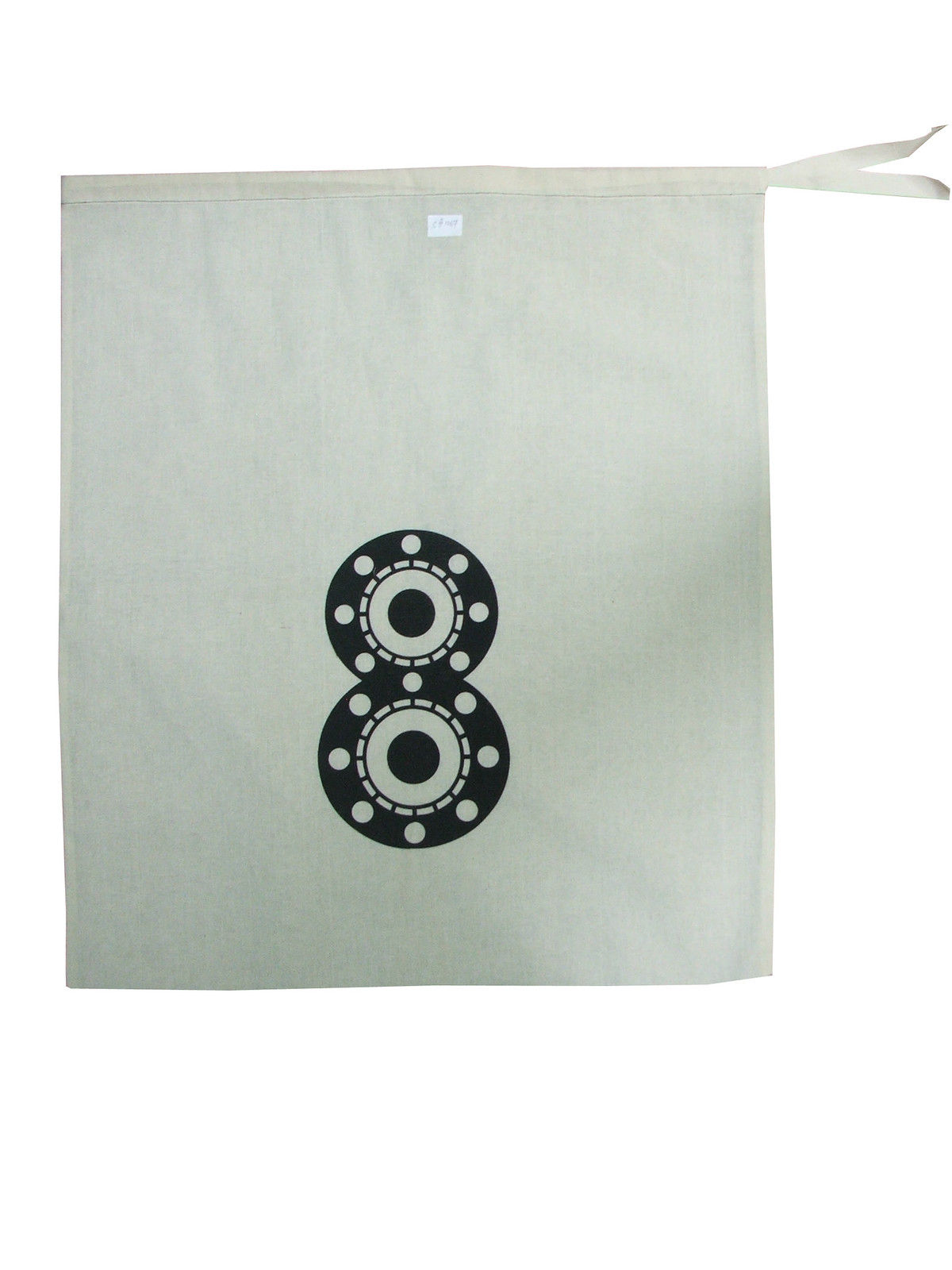The image depicts a light gray, rectangular pouch positioned vertically against a white background. At the top right corner of the pouch, two ribbons extend outward, resembling a drawstring that can be tied or pulled to close the bag. Directly beneath this narrow band, there is a small white square, possibly containing tiny, illegible writing. The most distinctive feature is the decorative numeral eight towards the bottom center of the pouch, formed by two black circles positioned one above the other. These circles each contain eight smaller white circles along their borders, which in turn have segmented edges resembling small bricks, and are centered around an inner black circle. The overall black-and-white palette of the pouch is complemented by subtle shadows, suggesting a slightly tinted color photograph.